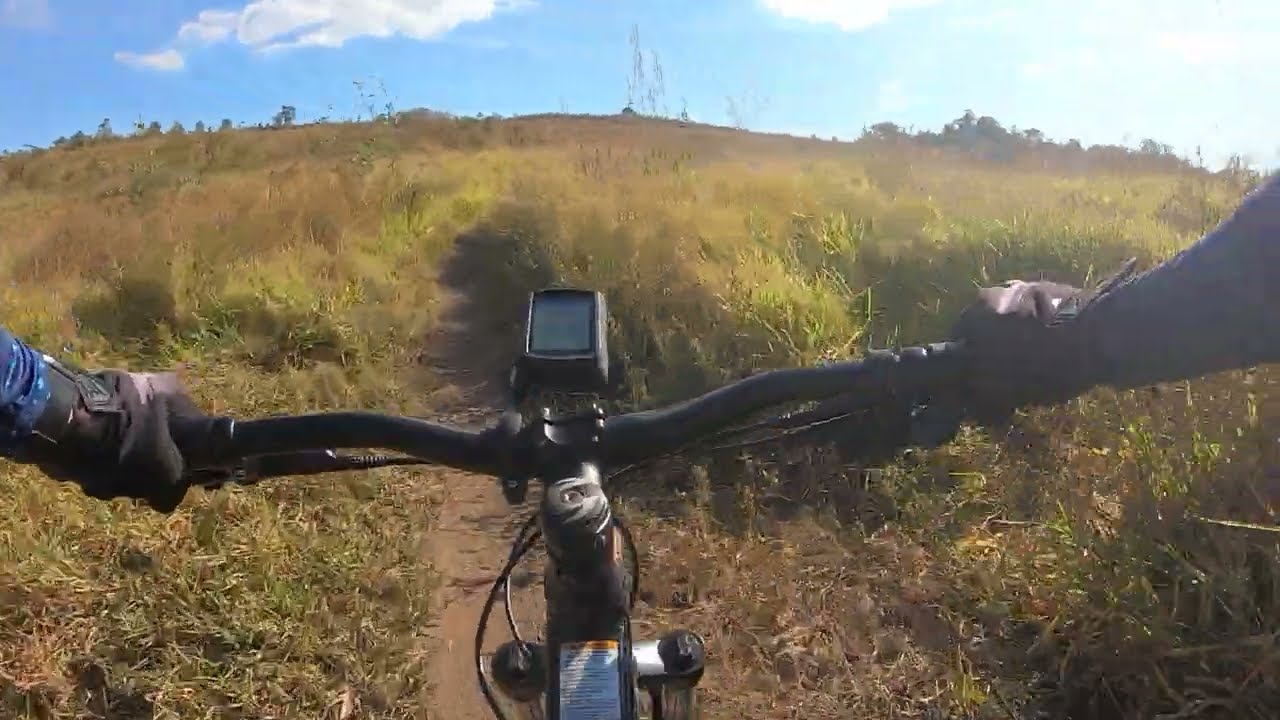The image captures the first-person perspective of a cyclist riding up a hill on a dirt path flanked by tall green and yellow grasses and bushes. The cyclist's black handlebars are gripping the foreground, with black-gloved hands visible, the gloves secured with Velcro straps. The sleeves of the cyclist's dark blue shirt are partially visible as well. At the center of the handlebars, a device—presumably for navigation or speed tracking—is mounted and readable by the cyclist. The path ascends the hill, dotted with sparse, thin trees along its crest. The sky above is light blue, adorned with puffy white clouds towards the top left, while the right side is bathed in brighter, whitish sunlight. Some electrical towers can also be seen in the distance atop the hill, mingling with the green and beige hues of the landscape.